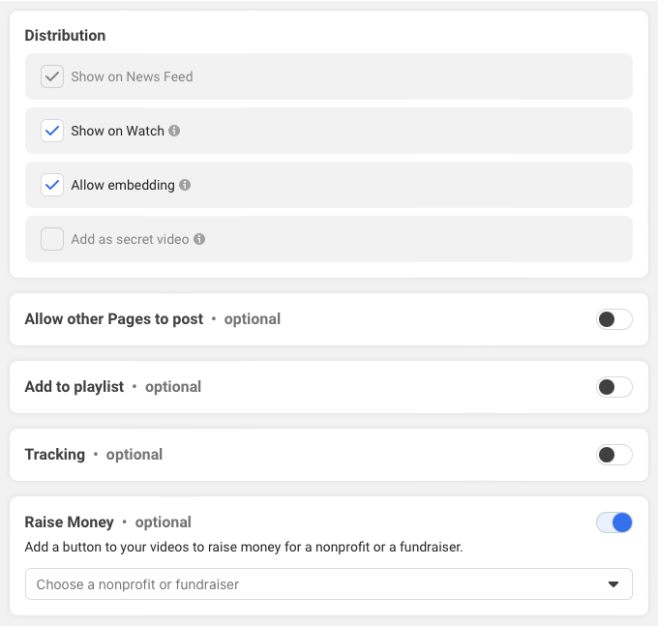The image is a screenshot from a website with a light gray background. Overlaying this is a white section at the top featuring a labeled rectangle with the heading "Distribution" in black text. Below this header, there are four selectable options, each accompanied by a small square checkbox. The first three options are checked, while the last one is unchecked.

1. "Show on Newsfeed" is checked with a gray checkbox.
2. "Show on Watch" and "Allow Embedding" both have blue checkboxes indicating they are enabled.
3. "Add as Secret Video" is unchecked, with an empty checkbox.

Further down, another white banner lists several additional options, each followed by the text "optional" and currently turned off:

- "Allow Other Pages to Post" (tooltip: optional)
- "Add to Playlist" (tooltip: optional)
- "Tracking" (tooltip: optional)
- "Raise Money": A detailed explanation follows, "Add a button to your videos to raise money for a non-profit or a fundraiser," accompanied by a dropdown menu to choose a non-profit or fundraiser. This option is highlighted in blue, meaning it is enabled.

The screenshot provides a detailed overview of options available for managing video distribution and additional functionalities on the website.